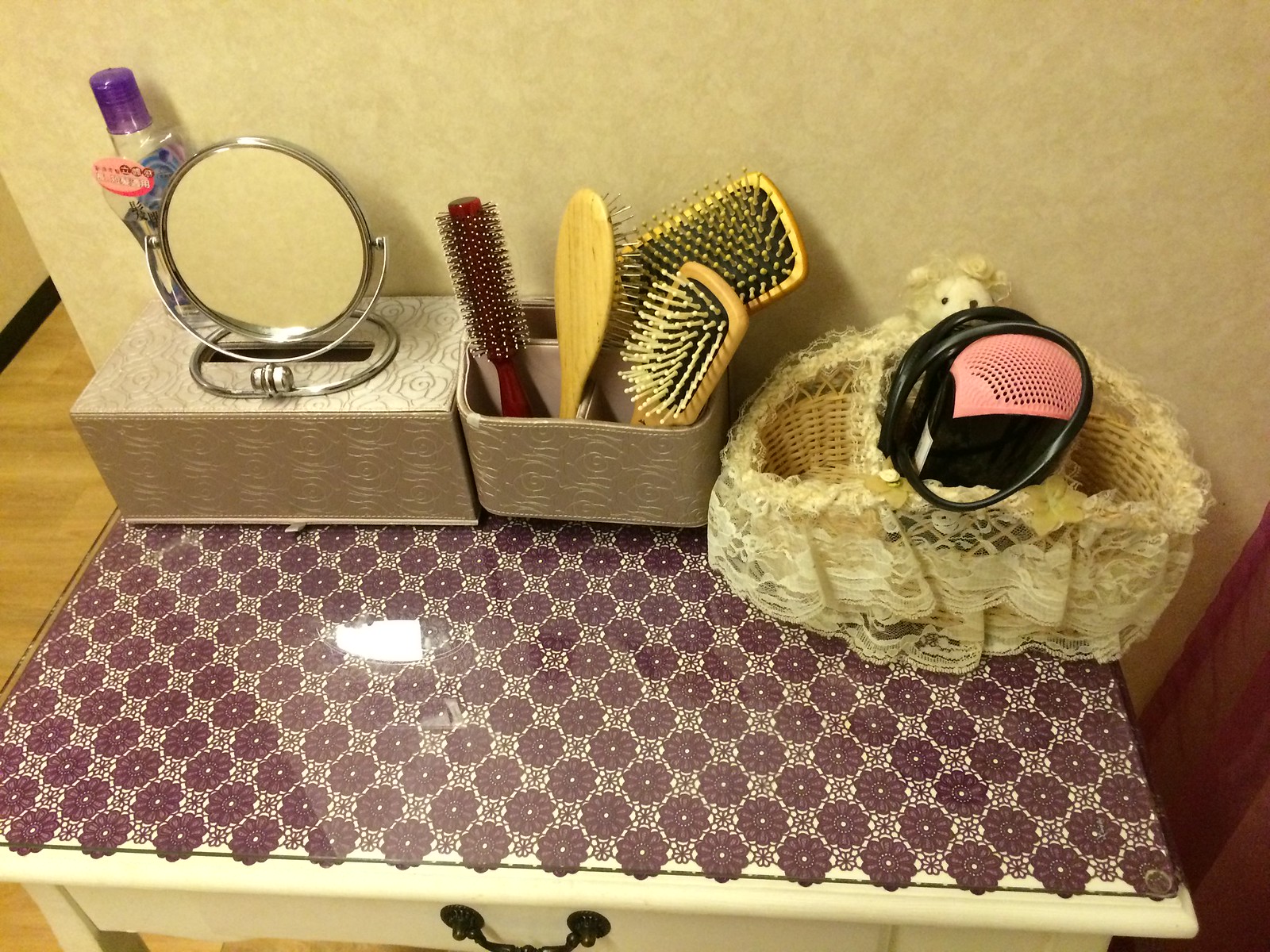The image depicts a white coffee table with a single drawer adorned with a black handle, positioned against a cream-colored wall near the room's corner. The floor features wooden planks complemented by black baseboards. The tabletop is decorated with a dark maroon floral pattern, possibly printed or encased in glass, with a crochet-like appearance. 

Three containers are neatly arranged on the table. On the far right is a pale wicker basket draped with a lace doily, holding a black and pink hairdryer neatly wrapped. In the center, there is a silver, embossed metal caddy divided into four sections, each holding a different hairbrush. The hairbrushes vary in shape and size, including a flat, wide rectangle, a shorter, thinner rectangle, an oval brush with wire and plastic bristles, and a dark red, round hairbrush with white bristles. Lastly, on the left, rests another silver box embossed with roses, resembling a Kleenex box cover, though it lacks tissues. 

Beside this box is a circular silver hand mirror, featuring dual magnification options, and seemingly placed behind it is a bottle of hair oil designed to manage frizz.